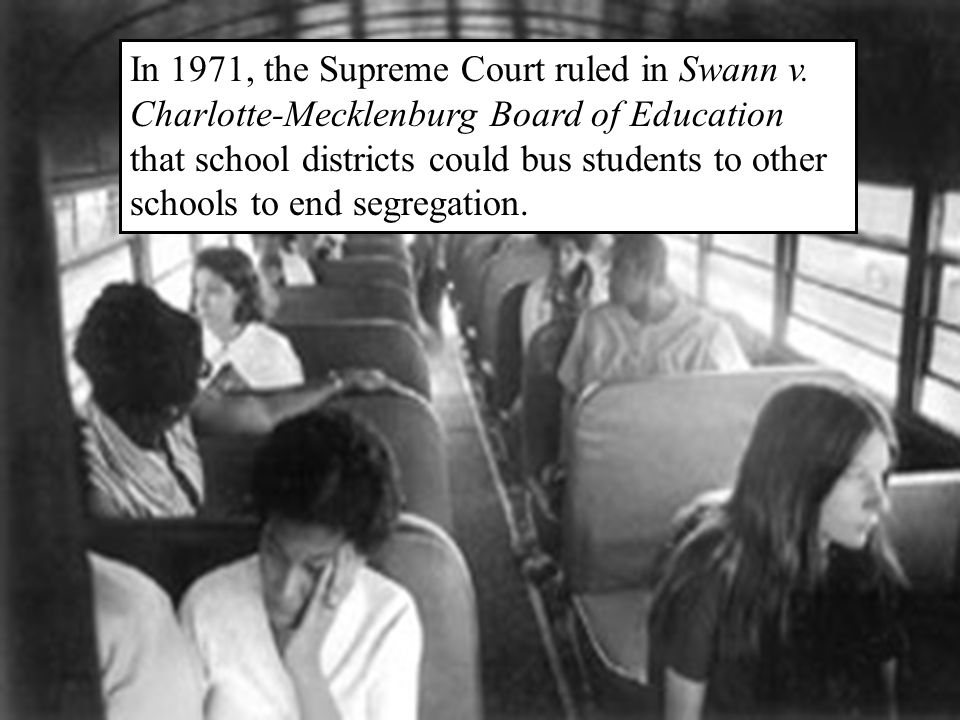This black and white image depicts a group of school children riding a bus, capturing a poignant moment in the history of school desegregation. The bus features rows of seats with an aisle down the middle, where the seating arrangement includes two children in the front seat on the left, and one child per row in the remaining seats on both sides of the aisle. The children are a mix of black and white students, reflecting the diversity achieved through school busing to end segregation. Some children appear lost in thought, staring out the windows, while one child is engaged in conversation and another rests their head in their hands. At the top of the image, a white rectangular box with black text, framed by a black border, reads: "In 1971, the Supreme Court ruled in Swann v. Charlotte-Mecklenburg Board of Education that school districts could bus students to other schools to end segregation." This caption emphasizes the significance of the 1971 Supreme Court ruling in combating the entrenched racial segregation in American schools during the Jim Crow era.